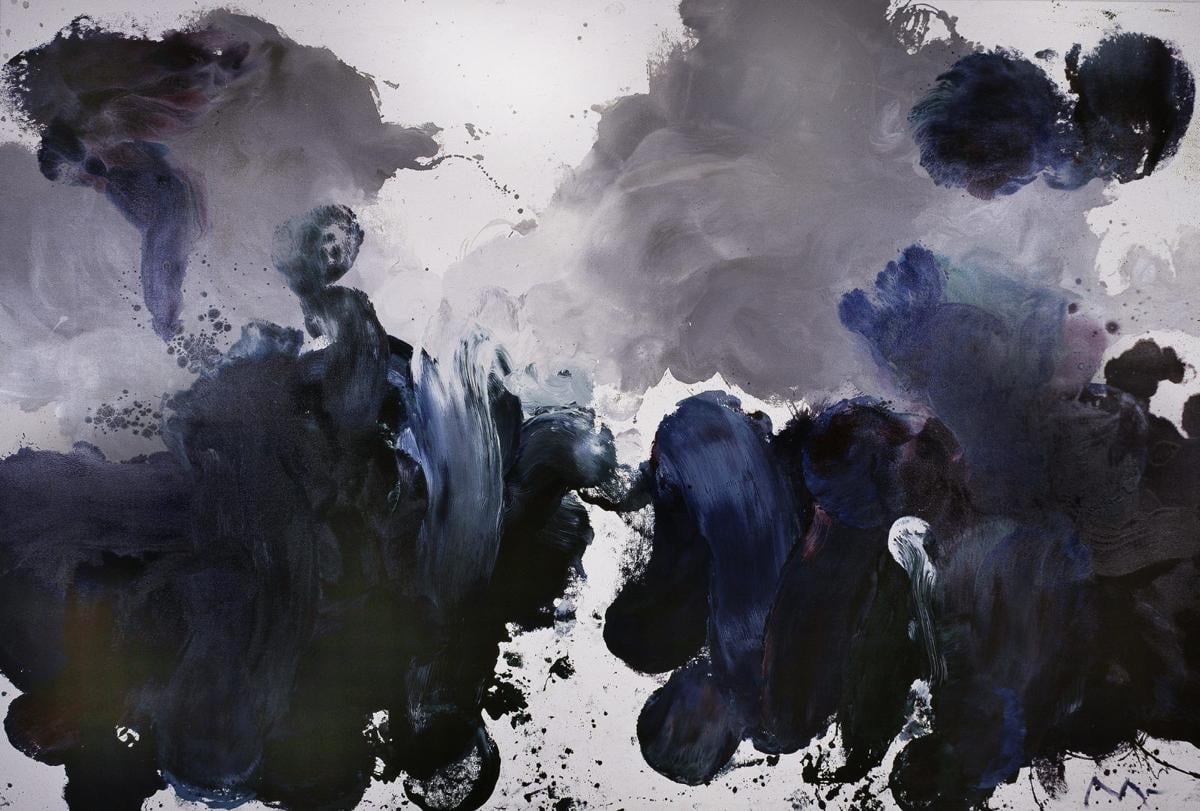This abstract painting features a large canvas with a predominantly grayish-white background. The composition includes dark blue paint applied in swirling, circular motions, mingled with gray and hints of white. The upper sections and both the right and left edges host numerous fluffy, cloud-like forms, created through similar swirling brushstrokes that give the artwork a textured, three-dimensional appearance. Notably, two dark blue, pom-pom-shaped blobs are positioned in the top right corner, with larger, darker pools of blue paint concentrated towards the bottom. The piece exudes a dark and ominous atmosphere, reminiscent of an inkblot test, inviting viewers to interpret its abstract elements in their own way.